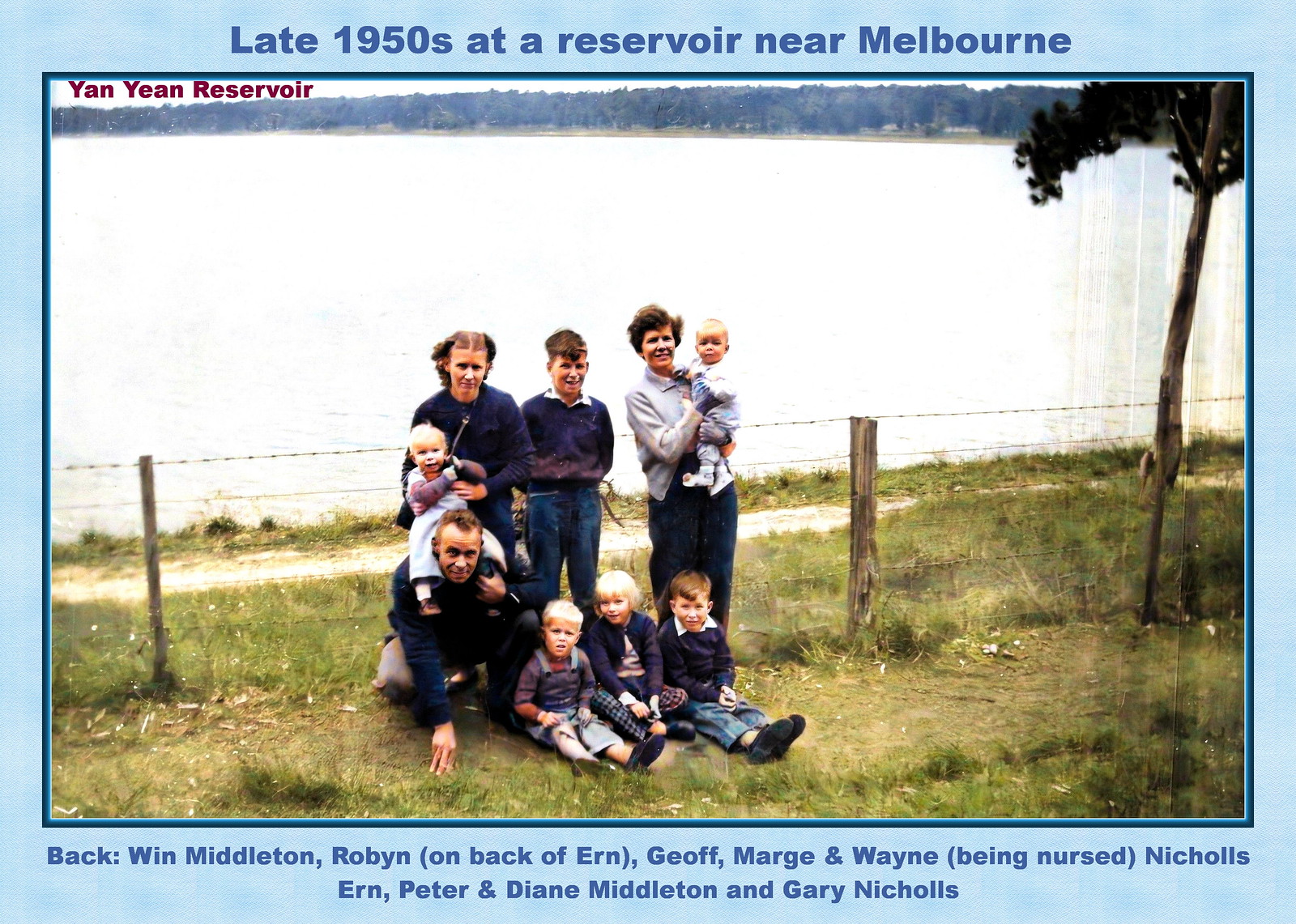This vintage color photograph, from the late 1950s, captures a family of ten members at the Yan Yin Reservoir near Melbourne. The photo is bordered by two blue edges: a narrow dark blue inner border and a wider light blue outer border. Above the image, in bold navy blue lettering, is the caption "Late 1950s at a Reservoir near Melbourne." Below the image, also in dark blue text, are the names of the family members: Beck, Wynne, Middleton, Robyn, (on the back of Erin), Geoff, Marg and Wynne (being nursed), Nichols, Ern, Peter, and Diane Middleton, and Gary Nichols.

The family is posing together on a green grassy area. The backdrop features a large water body—a reservoir—spanning across the width of the image with a metallic wire fence marking the boundary between the grass and the water. In the distance, the opposite shore is densely lined with trees. To the right, a solitary tree adds to the picturesque outdoor setting. The family includes a mix of adults, children, and babies, with three children sitting in front, some people standing, and two adults holding infants. The serene, daytime scene is anchored by the family's composed and happy demeanor.